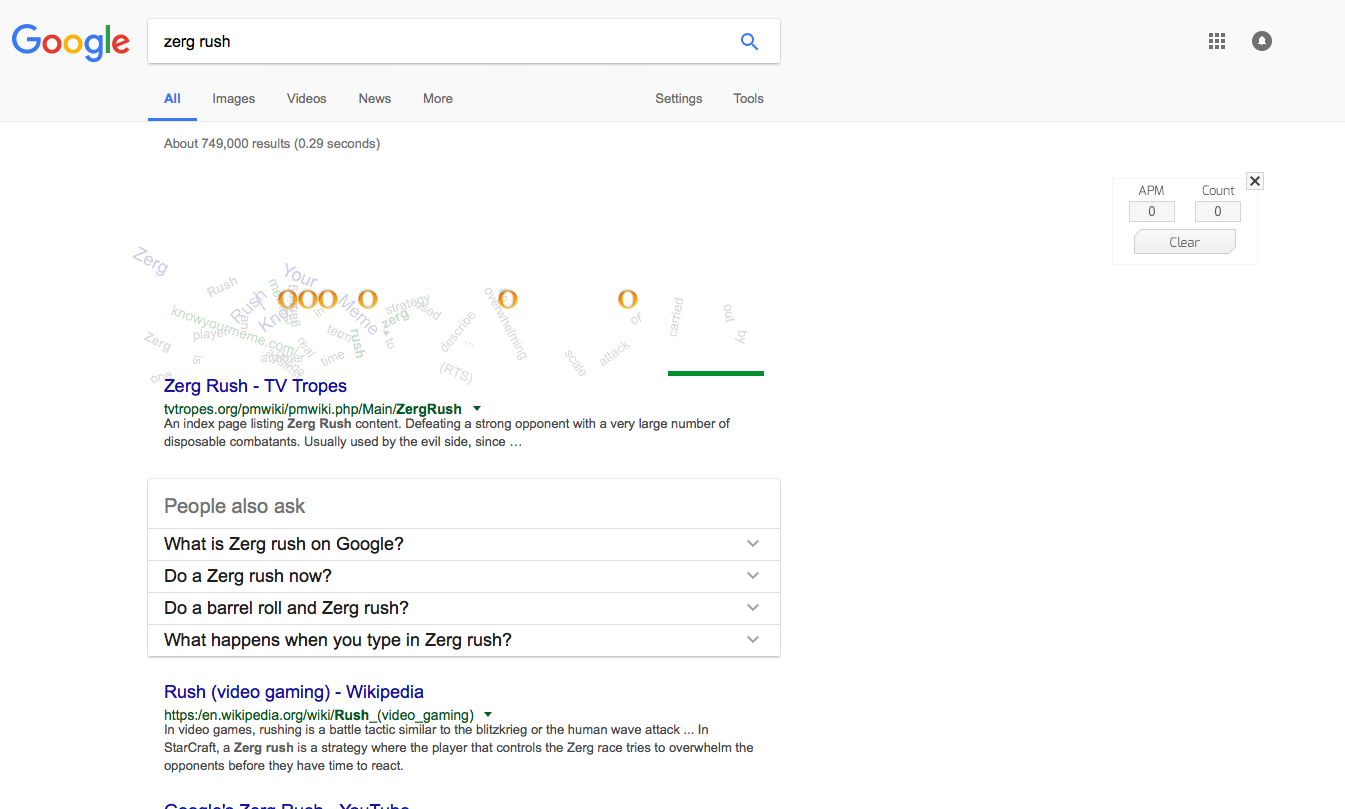A Google search for "Zerg Rush" reveals various resources detailing this gaming tactic, including a TV Tropes page that specifically lists content related to Zerg Rush. According to TV Tropes, Zerg Rush refers to a strategy where a large number of disposable combatants, typically from the evil side, are used to overwhelm the opponent. Commonly asked questions on Google about Zerg Rush include "What is Zerg Rush?", "Do a Zerg Rush now?", "Do a barrel roll on Zerg Rush?", and "What happens when you type in Zerg Rush?". Additionally, "Rush Gaming" mentions that rushing is a battle tactic in video gaming similar to blitzing or human wave attacks. In the game StarCraft, a Zerg Rush involves the player who controls the Zerg race deploying a rapid, overwhelming attack against their opponent before they can adequately prepare or respond. The small font on the screen makes it challenging to read the text clearly.